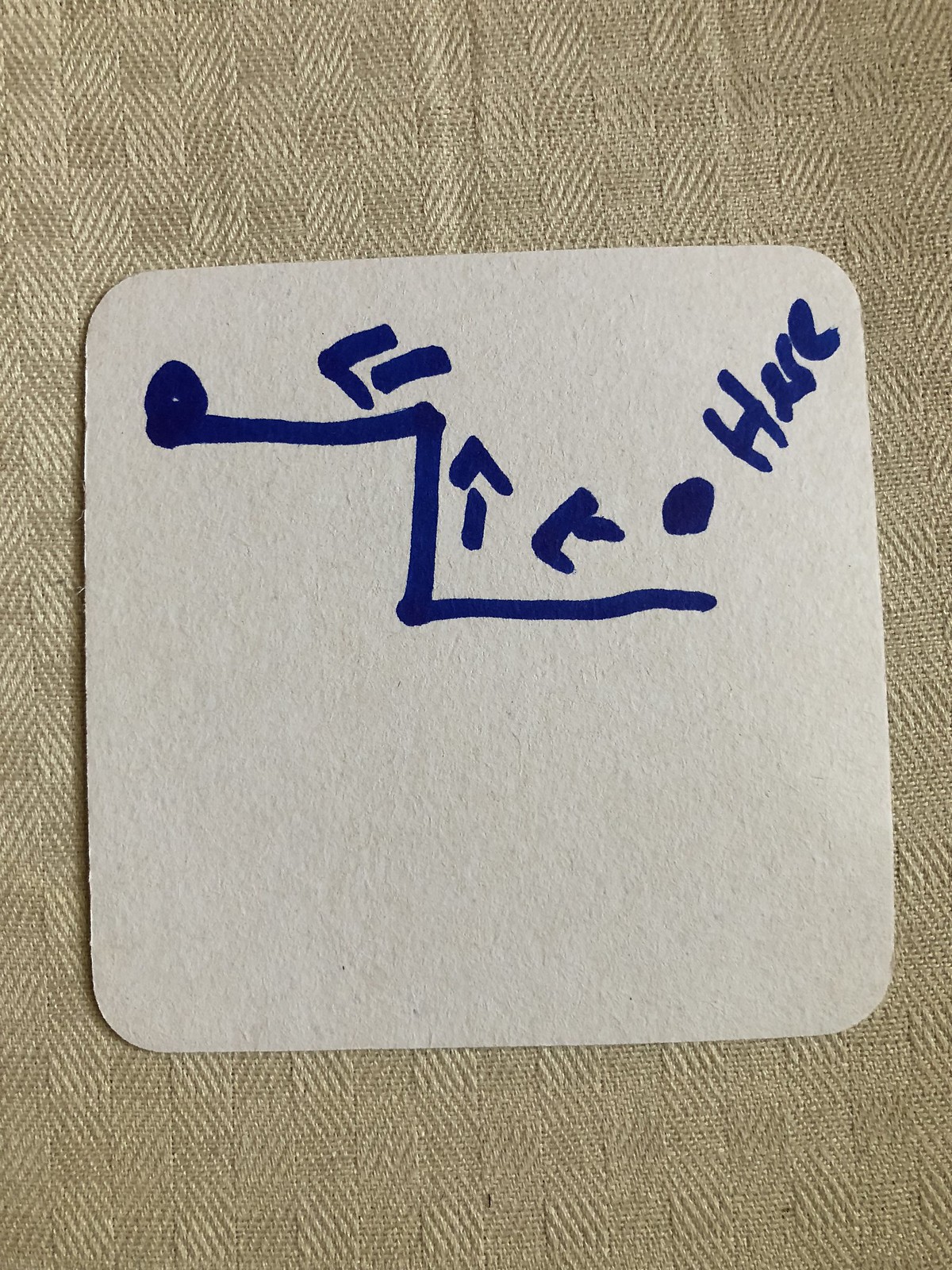In this image, a piece of greyish fawn fabric is featured prominently, woven into a pattern of tiny squares using taupe or beige-colored thread. The fabric is slightly askew, with the bottom right corner revealing incomplete squares, indicating it was not cut precisely along the warp. Centered on this fabric is a tilted white object, possibly card or a non-woven material like felt, which aligns more closely with the fabric's weave.

The white piece showcases an intriguing, roughly drawn diagram. In its upper half, there is a step and flat surface, with a circle positioned at the left end. An arrow head, with a dash before it, points towards this circle. Following this, the diagram continues down to the next step, accompanied by another roughly drawn arrow. The arrows are inconsistently drawn, with their heads not fully connecting to their stems. Additionally, there is a round blob near the drawing. Slightly tilted and resembling the letter "Z," the word "here" is inscribed, with a capital H and lowercase 'e-r-e,' positioned towards the right-hand corner as a directional marker. The entire image gives off a whimsical and somewhat mysterious vibe due to the unusual alignment and the crude sketchings.